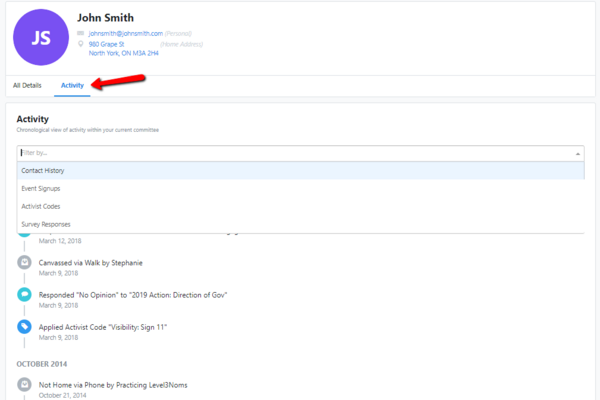The image depicts a detailed section of an individual's account profile. In the upper-left corner, there is a circular icon featuring a vibrant purple background with the white initials "JS" prominently displayed in the center. To the right of this icon, the name "John Smith" is written in bold black text. Directly beneath the name, "johnsmith@johnsmith.com" is listed as the email address, followed by the physical address "980 Grape Street, North York, ON M3A 2H4."

A red arrow points to a tab labeled "Activity." Below this tab, the heading "Activity" appears again. Below the heading, a search bar is available with the placeholder text "Filter by contact history, event signups, activists, codes, or survey responses." At the very bottom of the image, there is a date listed as "October 2014."